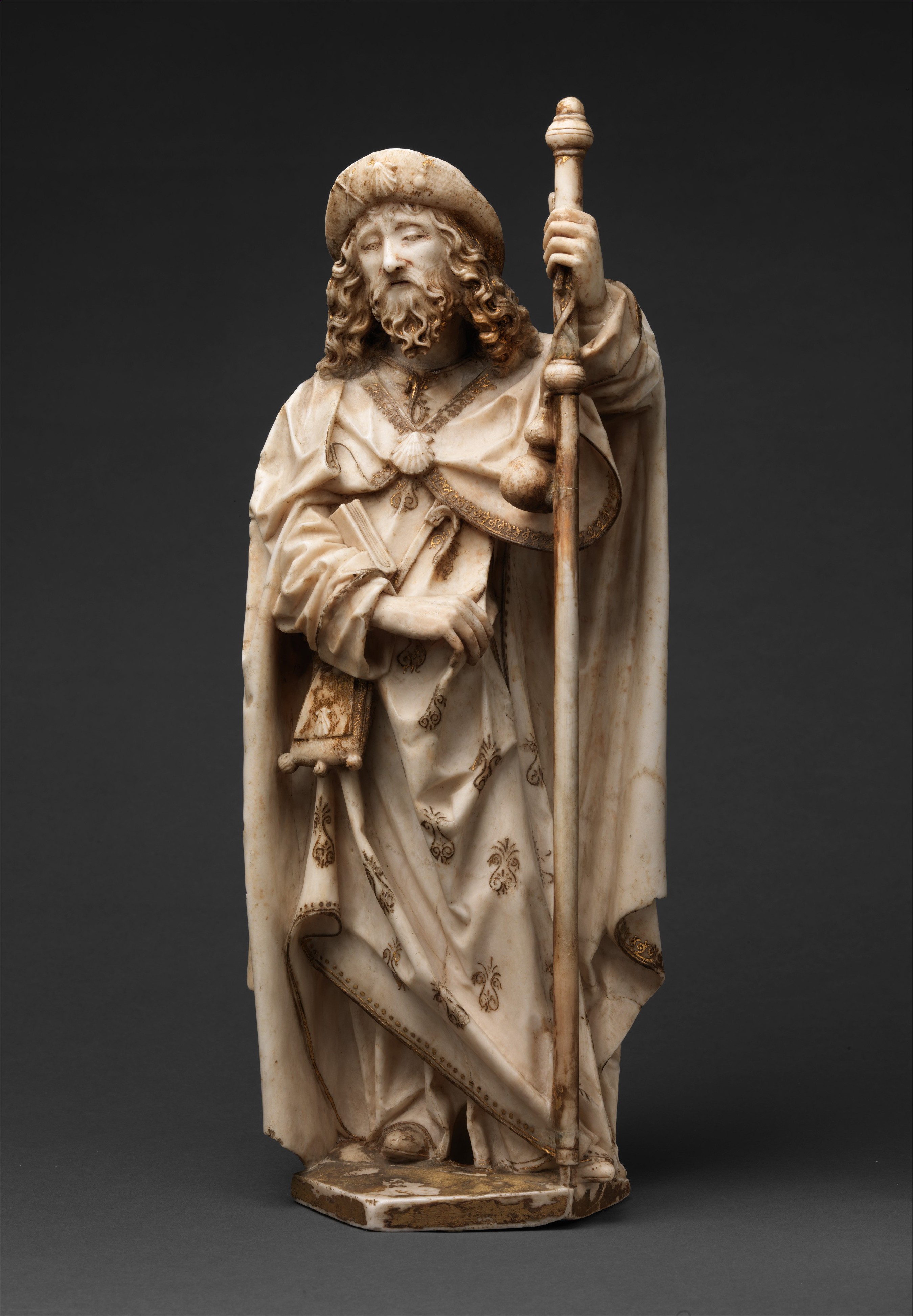The image showcases a ceramic figurine of a shepherd or wise man standing on a dark brown platform against a predominantly dark gray background, with the bottom part slightly lighter. The central figure is dressed in flowing, vintage robes with pineapple-shaped patterns in dark brown, featuring gilded fringes and a pin holding the outer cloak together. The figure is characterized by long curly hair, a beard, and a circular soft hat or turban, holding a long shepherd's staff in his left hand. The main colors of the statue are off-white with darker brown accents, and the figure’s eyes are peacefully closed, lending it an air of serenity.